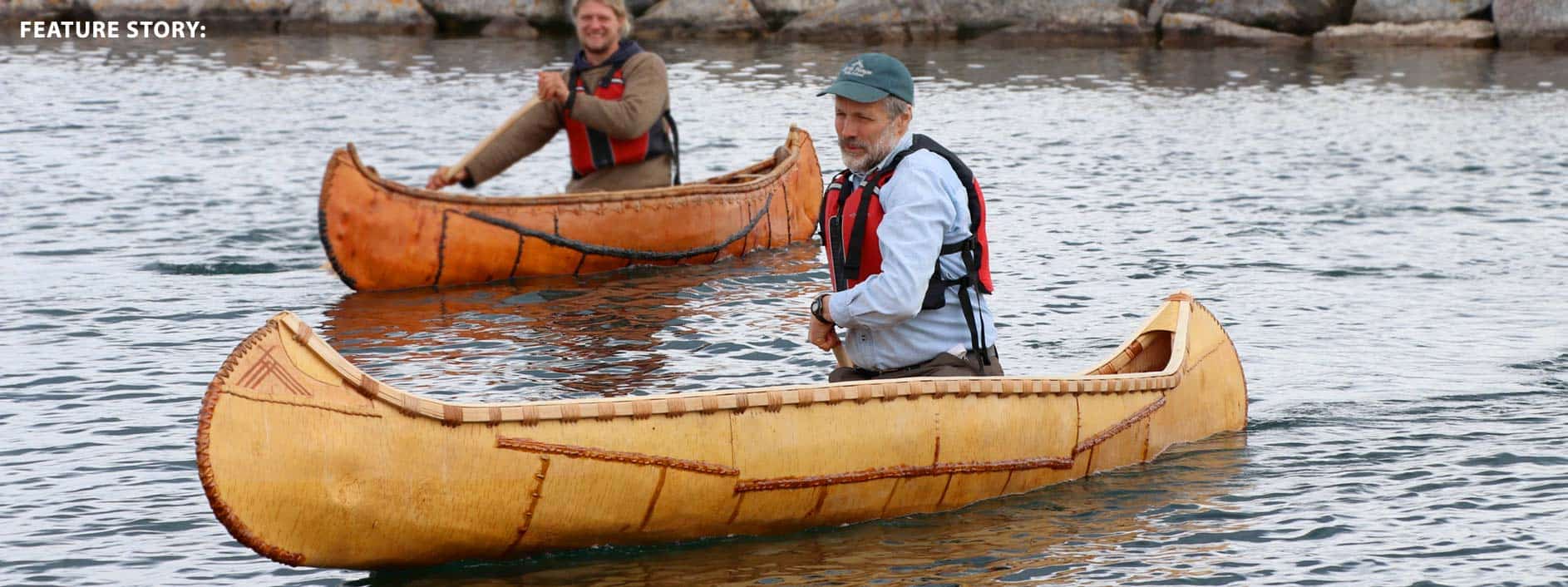The image is a detailed photograph capturing a scene likely from a documentary, featuring Jon Stewart and another man kayaking in separate canoes on a canal. Jon Stewart, identifiable by his white beard, wears a green hat, a blue shirt, and a red life vest, and is in a light tan kayak with medium brown stripes. The second individual, wearing a brown shirt and a red life vest, is in a dark, rusty brown kayak with black trim and slanted lines. Both are actively paddling. The backdrop includes a stone wall and a shoreline with large rocks, indicating their proximity to the shore. In the top left corner of the image, the text "Feature Story" is prominently displayed.